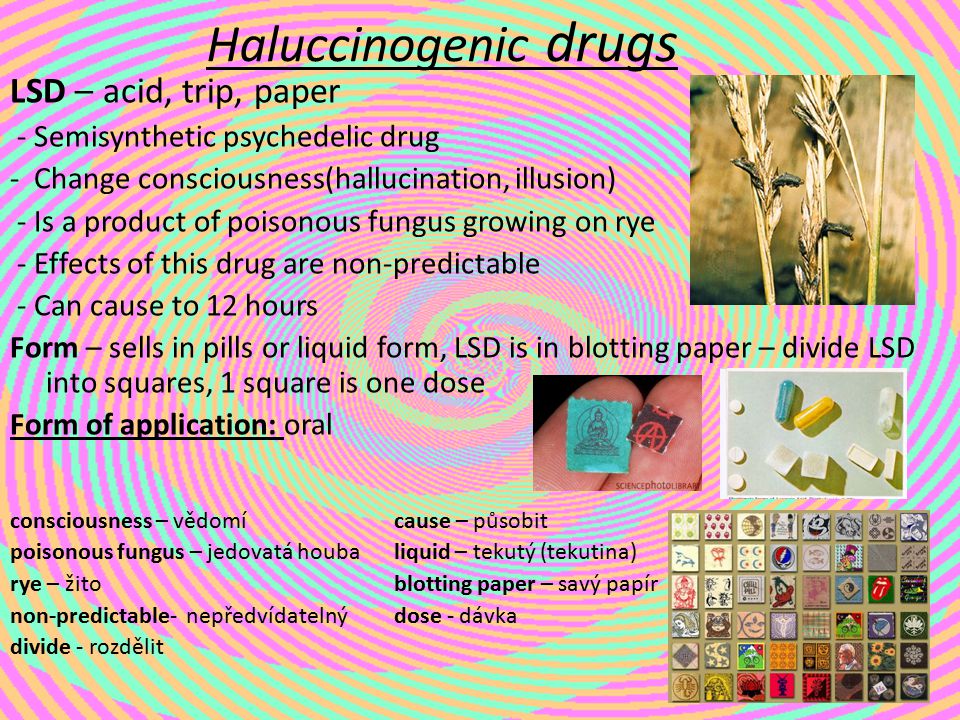The image appears to be a detailed informational slide from a presentation about hallucinogenic drugs, particularly focusing on LSD. It's horizontally oriented with a trippy background featuring an elongated spiral of vibrant, alternating stripes in blue, purple, subtle yellow, dark pink, and orange, which gives an illusion-inducing effect. 

At the top center in large, black, underlined text—it reads "hallucinogenic drugs," with only the 'H' capitalized. Below that, the slide features a textual breakdown: 

- "LSD" in bold, all uppercase followed by "- acid, trip paper."
- "Semi-synthetic psychedelic drug" and "Change consciousness (hallucination, illusion)".
- "Product of poisonous fungus growing on rye."
- It continues with information about the unpredictability of effects, which can last from 2 to 12 hours.
- Different forms of LSD are noted: cells in pills, liquid form, and blotting paper divided into squares, with one square equating to one dose.
- The form of application is specified as oral.

A glossary in two languages (one being English and presumably French or another European language) is neatly aligned towards the bottom, explaining drug-related terms such as "consciousness," "poisonous fungus," "rye," "non-predictable," "divide," "cause," "liquid," "blotting paper," and "dose."

On the right side, the slide is enriched with photographs: 
- A grid of LSD tabs, each adorned with different designs such as green spots, a red cartoon mouth, orange with black sections, and various symbolic and abstract patterns.
- Above the tabs are two smaller rectangles: one showing an assortment of pills on a light blue background and the other a pair of young fingers holding a rectangular LSD tab with a Buddha illustration.
- Above these, there’s an image depicting tan stalks of rye.

All textual information is meticulously organized and left-aligned, providing a comprehensive and visually engaging overview of LSD and related terminology, making it an informative piece likely from a slideshow presentation aimed at educating about these substances, potentially from the 1980s or 1990s.